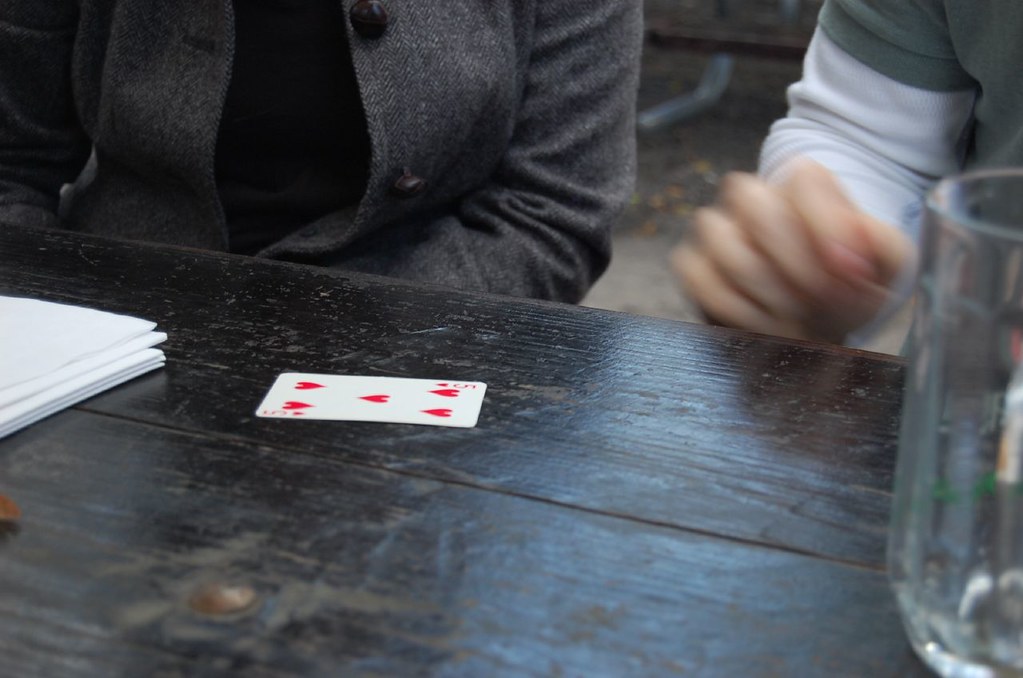This photo captures a close-up view from tabletop level, focusing on a weathered wooden table with a black finish. The table clearly shows signs of age, with distinct wood grains and a worn appearance. A rusty screw, part of the table's structure, has chipped away some of the surrounding paint, further emphasizing the table's vintage character. 

Prominently displayed on the tabletop is a single playing card, the Five of Hearts, oriented face-up. Adjacent to the card is a neat stack of white papers. To the side of the papers sits an empty glass, which appears to be a beer mug adorned with some insignia.

In the background, two men are partially visible from the arms down, their faces obscured. One man is dressed in an unbuttoned tweed jacket over a black shirt, while the other sports a green t-shirt layered over a long-sleeved white shirt. Their presence, though not fully seen, adds a human element to the scene, suggesting a pause in an ongoing activity.